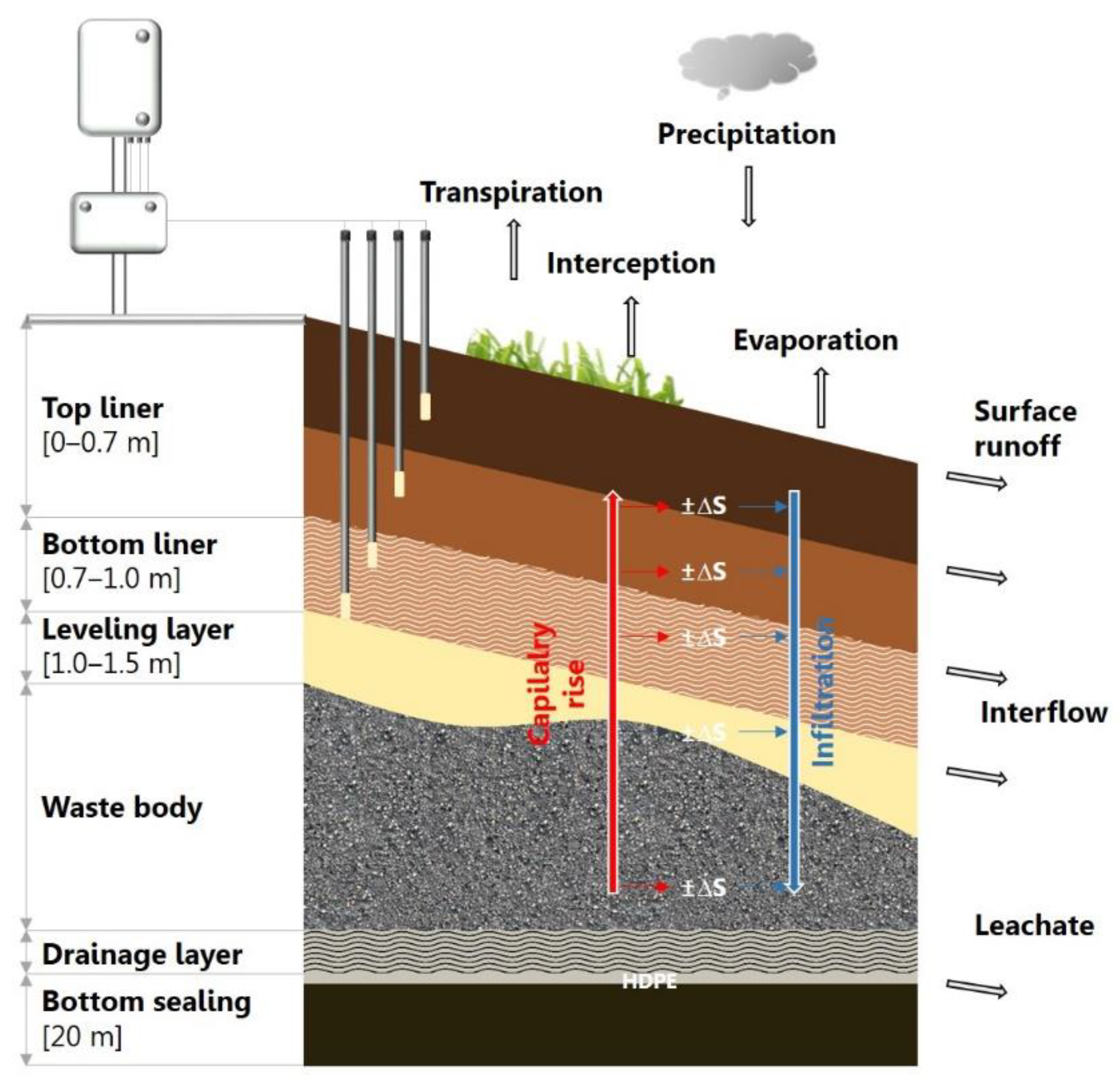This detailed illustration depicts an in-ground filtration system, demonstrating how water interacts with various soil layers. The diagram is oriented with text and arrows pointing to different processes involved in water movement, including precipitation, transpiration, evaporation, surface runoff, interflow, and leachate. The layered structure starts with a dark brown top liner, followed by a lighter brown bottom liner. Below that is the leveling layer, represented by a tannish color. Next is the waste body layer, depicted as gravel. Beneath this is the drainage layer, and finally, the bottom sealing layer, illustrated as a solid black bar. The text labels each layer to the left side, providing clarity on their composition and functionality within the system. This comprehensive diagram offers a visual explanation of how modern landscaping or urban development affects water flow and filtration through different soil layers.